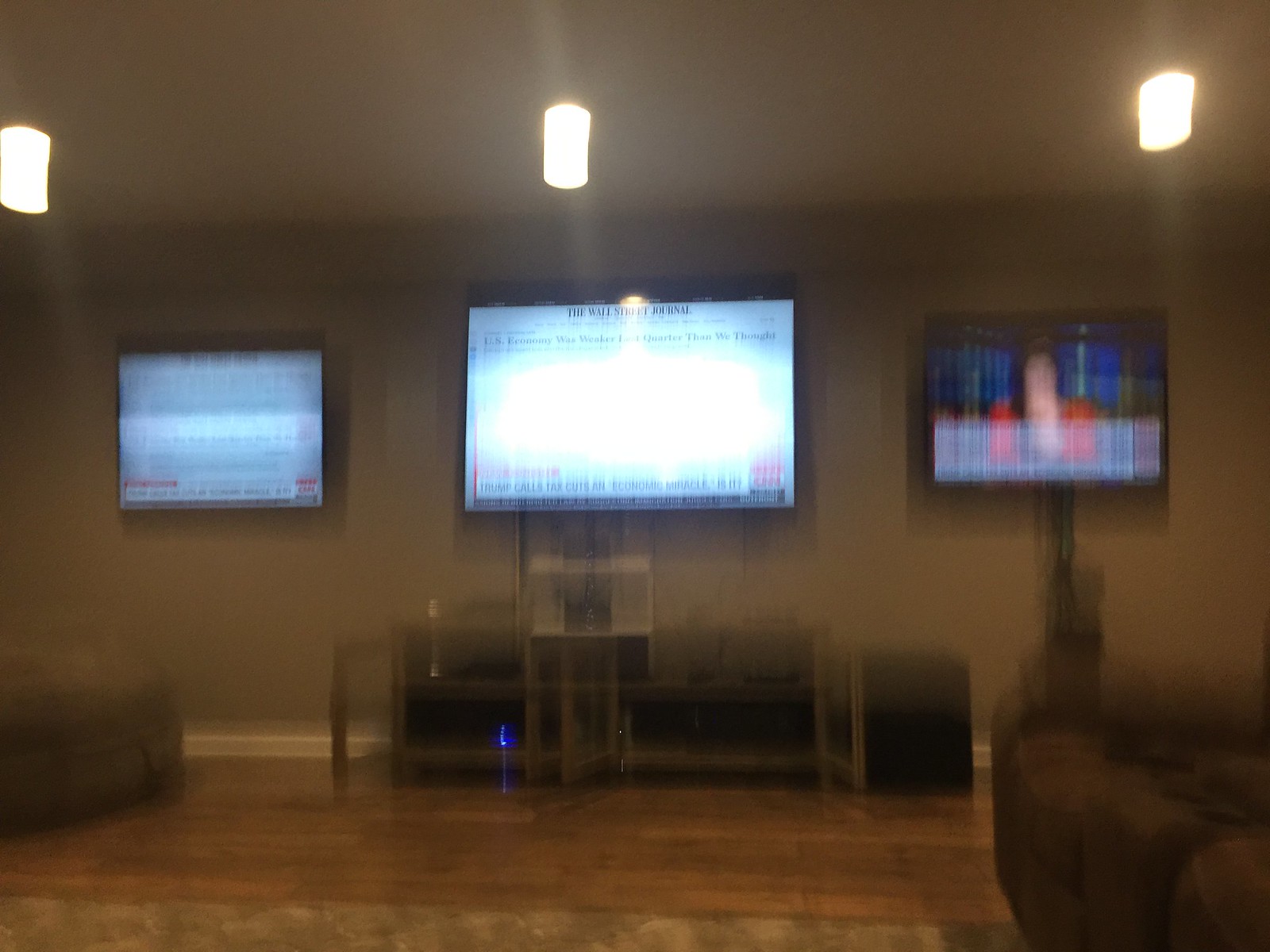The image is a very blurry photograph of a large living room or den, featuring three mounted TV screens on a light brown wall. The center TV is the largest and displays text, with "The Wall Street Journal" faintly visible at the top. Surrounding it, the left and right TVs are smaller, with the right one showing a woman in red against a bluish background. Below the center TV, there's an entertainment cabinet with shelves, possibly holding equipment and storage. Positioned in front of the setup is a central table, with a brown cushion chair to the left and a couch chair to the right. The room has three hanging lights on the ceiling, casting a glow over a brown and slightly green rug on the floor. Additional features include a hardwood floor, and hints of other furniture potentially for storage or seating, contributing to the overall sense of a spacious but indistinct rec room.